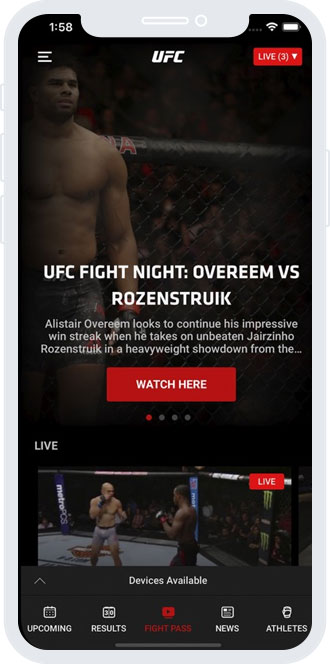A person is closely examining the UFC webpage on their phone, with a visible battery life and strong Wi-Fi signal at the top. The header shows "158," flanked by the UFC logo in white. To the left is a three-line menu icon, and to the right, a live indicator with "3" in parentheses. Below this is a red dropdown box.

In the center of the screen, there's an image of a muscular fighter in the ring, wearing small shorts and sporting short hair that suggests a mixed heritage. The banner reads "UFC Fight Night: Overeem vs. Rozenstruik." Below, it states, "Alistair Overeem looks to continue his impressive win streak when he takes on unbeaten Jairzinho Rozenstruik in a heavyweight showdown." There's a red "Watch Here" button.

A red dot along with three others indicate a carousel of related UFC content. Below, there's a live video feed showing two fighters in the octagon about to face off. The screen also displays "Device Available" in white text, along with options for "Upcoming Results" and "Fight Pass," both highlighted in red. At the bottom, there are tabs for "News" and "Athletes" for further exploration.